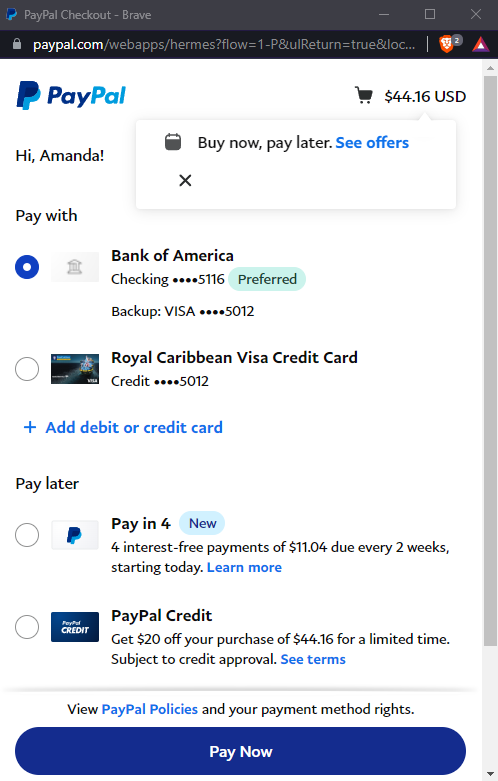This is a detailed screenshot of a PayPal checkout page viewed on a tablet in the Brave browser, indicated by the text "PayPal checkout - Brave" at the top. The interface displays a vertical orientation, suggesting a larger screen than a cellphone.

The URL bar shows "PayPal.com," and below it is the recognizable PayPal logo, featuring a dark blue and electric blue color scheme with a 'P' overlaid on another 'P'. On the right side, there's a shopping cart icon and the total cart amount, $44.16 USD. Adjacent to this is a pop-up offering the option to "Buy now, pay later" or view offers, which can be closed with an 'X'.

Under the logo, a personalized greeting reads "Hi Amanda," followed by the payment section. Amanda is presented with multiple payment options:

1. **Bank of America Checking Account** (marked as preferred), with a backup Visa card linked to it.
2. **Royal Caribbean Visa Credit Card**, showing the last four digits of the card number.

Additionally, there's an option to add a new debit or credit card.

Further down, Amanda can choose a "Pay Later" option, which offers two plans:

1. **Pay in 4**: Four interest-free payments of $11.04 due every two weeks, starting today, marked with a "NEW" tag.
2. **PayPal Credit**: Receive $20 off the purchase of $44.16 for a limited time, pending credit approval.

Concluding the page is a prominent blue "Pay Now" button, finalizing the checkout process.